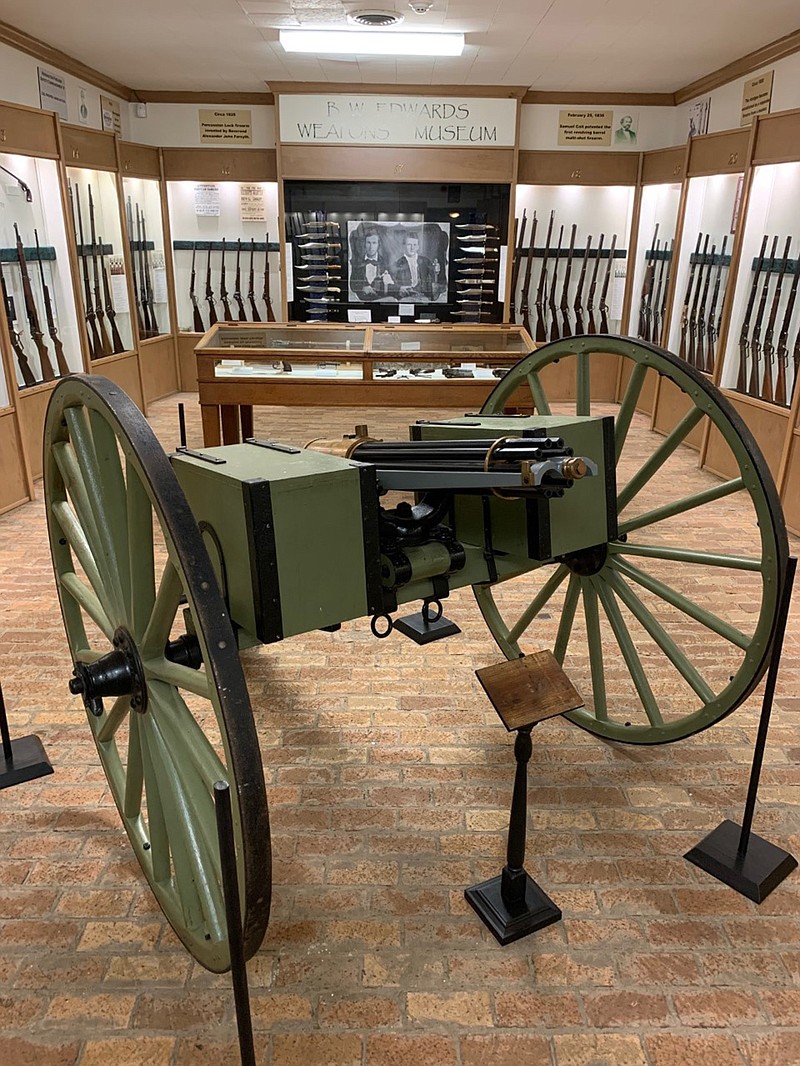The image captures an exhibit within the B.W. Edwards Weapons Museum, focusing on a green cannon with black wheels prominently positioned front and center. The cannon, primarily green with black accents, draws immediate attention in the room. Surrounding the cannon, the side walls and portions of the back wall are adorned with various types of weaponry displayed on gun racks, showcasing an extensive collection of historical arms. The middle section of the back wall features a black display space housing a photograph of two men clad in suits. Flanking this photograph is a well-arranged assortment of knives. Above the black display space, a white sign with black lettering proudly announces "B.W. Edwards Weapons Museum." Directly in front of this backdrop is a brown wooden display case, though its contents are obscured from view due to the angle at which the photograph was taken.